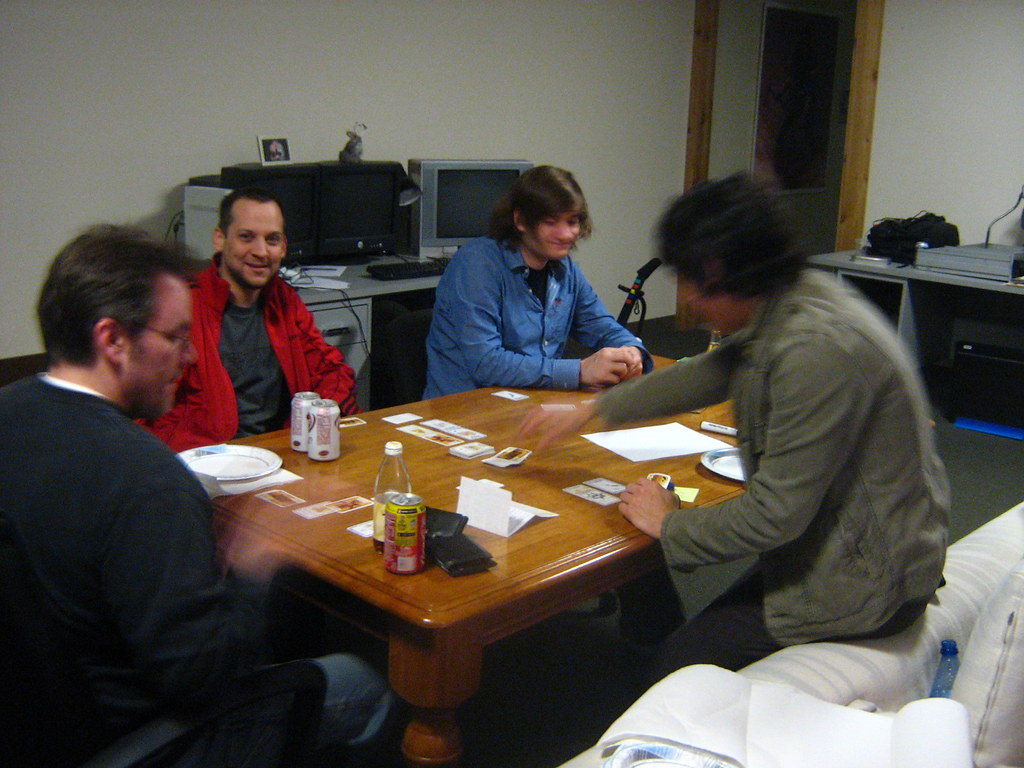This color photograph captures a lively scene of four middle-aged Caucasian men engaged in a card game, seated around a table in a somewhat cluttered room. The room is furnished with various desks, a dated box-style TV, and a computer. Scattered around the table are three soda cans, a glass bottle, two white paper plates, several cards, and wallets. 

In the foreground to the left, a man wearing a black sweater over a white shirt, with glasses and short hair, is in mid-movement, making his hand appear blurry. To his right, another man with an olive green jacket and dark hair reaches for a card, his image slightly blurred. 

In the background to the left, a man with a bright red jacket over a gray shirt, short-cropped hair, and a goatee, looks directly at the camera with a smirk. Next to him, a man with medium-length shaggy brown hair, wearing a blue button-down shirt, looks down at the table, smiling, with his hands clasped together. The overall ambiance suggests a casual, friendly gathering, amidst a mix of modern and slightly dated electronic devices.